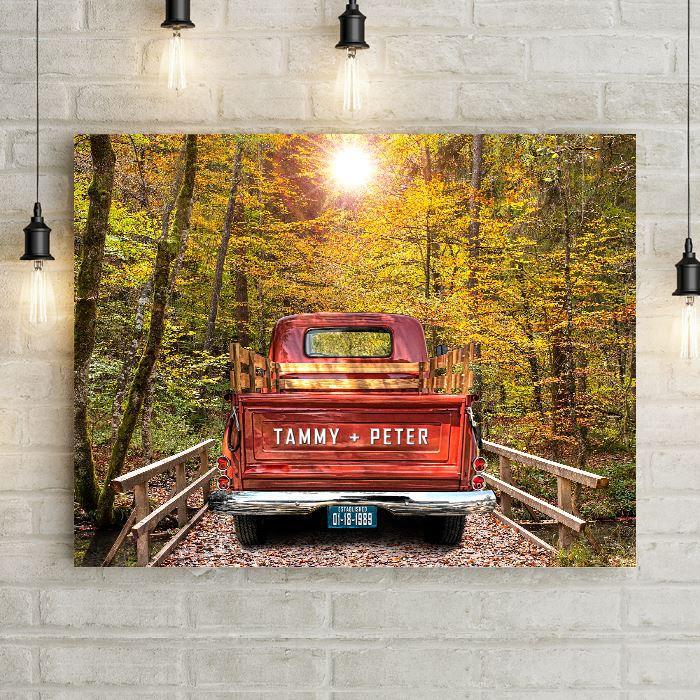The image depicts an old red pickup truck with an open bed, built up on the sides with wooden boards. It is parked on a small wooden bridge covered in autumn leaves in varying hues of orange, yellow, and red. On the tailgate of the truck, which is facing away, "Tammy + Peter" is inscribed in white capital letters, and beneath it is a blue license plate with white text, displaying the numbers "01181989." The bridge is surrounded by dense woods with colorful fall foliage, and the bright white sun is shining down, casting rays over the scene. This entire picturesque scene is captured in a photograph hanging on a white brick wall, illuminated by black light fixtures with long strings, enhancing its display.